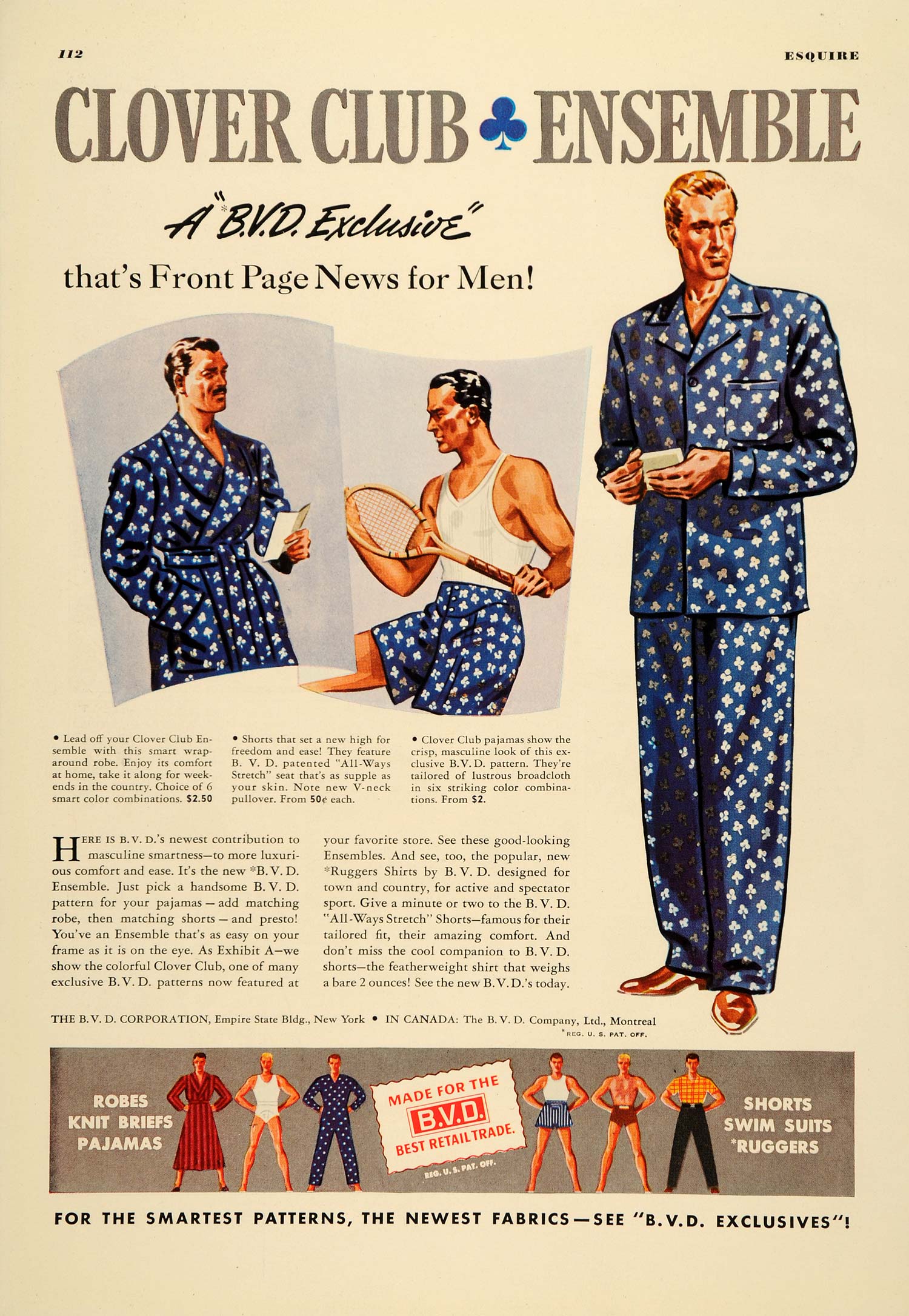This image is a full-page advertisement from an old issue of Esquire magazine, specifically page 112 as noted in a small black font in the upper left corner. The magazine's name, Esquire, appears in a small serif font in the upper right corner. Dominating the page is a large header in dark gray text that reads "Clover Club Ensemble," with a blue clover symbol placed between the words "Clover" and "Club." Below the title, handwritten black text states, “A BVD Exclusive. That's front page news for men.”

The advertisement features three illustrated men in stylish loungewear. On the left side, a man is depicted in a dark blue robe adorned with a white clover pattern. This same pattern is seen on the shorts of the man in the center, who pairs them with a white tank top and holds a tennis racket. To the right, a tall, lean man with slicked-back blonde hair wears a full dark blue pajama set featuring the same clover motif. The men are portrayed confidently, standing with their hands on their waists, exuding a sense of style and leisure.

Beneath these illustrations, there are captions with details and prices of the clothing items. At the bottom of the page, a gray banner showcases various men modeling different garments accompanied by a description stating, "Robes, knit briefs, pajamas, shorts, swimsuits, ruggers—made for the BVD Best Retail Trade.” Additional text at the bottom emphasizes, “For the smartest patterns, the newest fabrics see ‘BVD Exclusives.’”